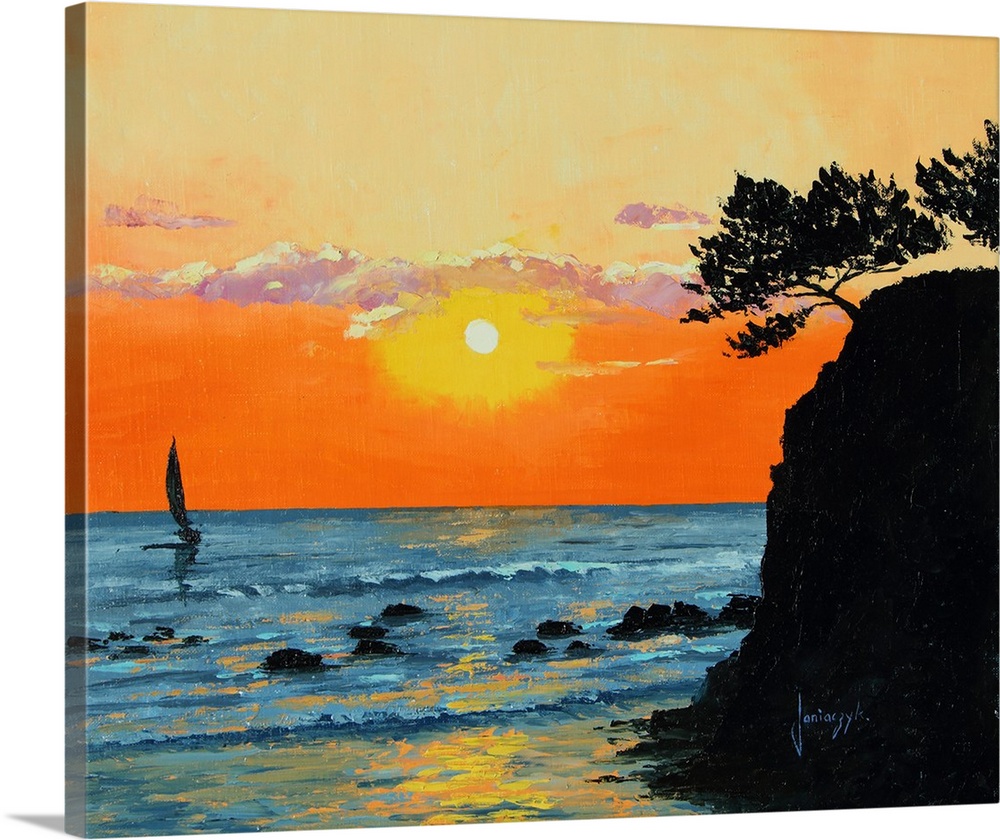This photograph captures a painting that has been slightly tilted, likely using a graphics editor, and placed against a white background, possibly as part of a mock-up for selling printed versions of paintings on canvas. The painting itself depicts a tranquil beach scene dominated by the ocean at the bottom. To the right, there is a prominent black silhouette of a cliff adorned with a couple of trees, one of which angles over the water. The sun in the distance glows intensely white, surrounded by gradients of yellow and orange, creating a vibrant sky with hints of purple hues and white highlights amidst some clouds.

In the water beneath, the bright reflections of the sun blend with various shades of blue, while black rocks punctuate the scene, with waves breaking around them. The silhouette of a small sailboat is visible in the lower-left part of the painting, adding to the serene atmosphere. The painting has a somewhat abstract and not overly realistic style, characterized by splotches of paint that suggest rather than define forms.

Finally, the artist's signature appears in the bottom right corner, inscribed in a light bluish color, though it is somewhat difficult to decipher, resembling "J-A-N-I-A-C-G-Y-L-S."